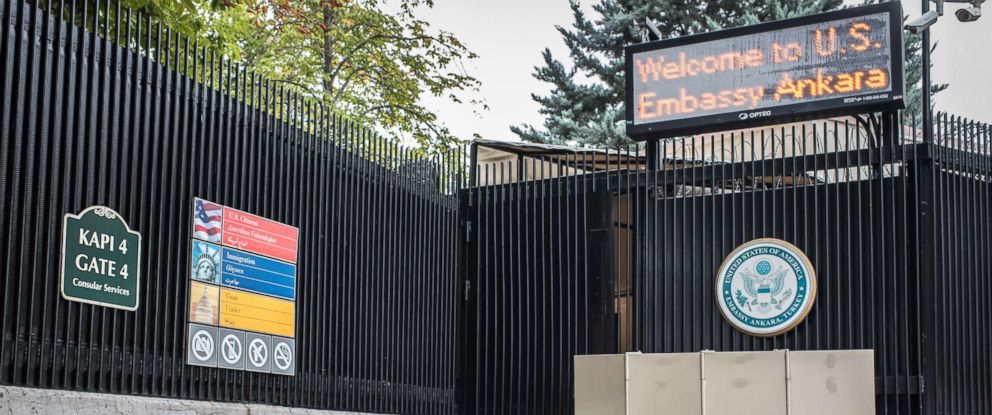This detailed image captures the exterior of the U.S. Embassy in Ankara, showcasing a wide shot of the black metal gate adorned with various signs and emblematic symbols. Dominating the gate is a prominently displayed digital sign that reads, “Welcome to U.S. Embassy Ankara.” The gate is sectioned horizontally and vertically, marked by a less welcoming appearance with symbols indicating prohibitions such as no photos, no cameras, and no smoking.

To the left, a green sign with white border and text reads “KAPI 4” and “Gate 4,” indicating an entry point. Next to this is a rectangular sign divided into three color segments. The top segment in red displays an American flag and white text; the middle segment in blue features the Statue of Liberty and more unreadable white text; and the bottom segment in yellow contains an image of the U.S. Capitol with brown text. Below these is a gray section with additional symbols constrained by circles with slashes through them, reinforcing restrictions.

Adjacent to this sign, a round emblem representing the United States is visible, rendered in green and white. Above the fence line, the tops of several trees, including both pine and regular varieties, are visible, adding a touch of nature to the scene along with a partial view of a white building in the background. A gray barricade occupies the bottom portion of the image, further contributing to the secure and fortified appearance of the U.S. Embassy's entrance.